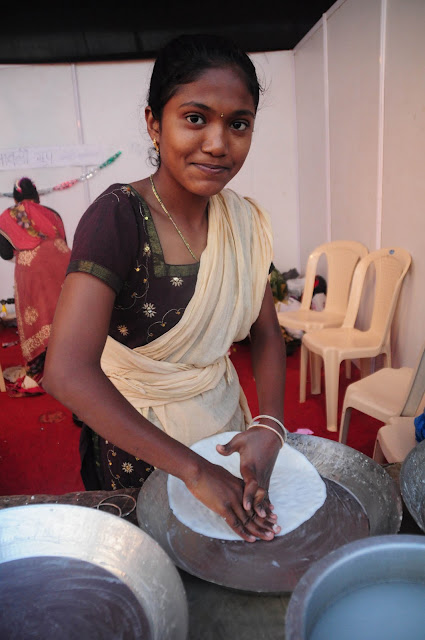This vertical color photograph captures a vibrant and engaging scene centered around a smiling woman of dark skin in a culturally rich setting. She stands confidently against a white wall with a contrasting black ceiling, immediately drawing the viewer's attention to her bright presence. Dressed in a striking dark purple dress adorned with green embroidered trim and delicate daisies, she epitomizes grace. A thin cotton cloth is elegantly draped around her shoulder and waist, adding to her traditional attire.

Her hands are actively engaged with a white circular piece of food or dough on a metal shelf behind her, which is lined with large, low metal bowls featuring wide rims. One hand presses against the dough while her other hand rests atop, showcasing a serene focus on her task. Her wrists are decorated with two bangles each, adding to the subtle yet beautiful details of her ensemble. She also wears a gold necklace, complementing her look.

To her left, another woman in a long red dress faces the back wall, providing a sense of depth and an insight into the communal activity. Behind the central figure, light yellow or off-white plastic chairs line the wall below colorful streamers, suggesting a festive environment. A red carpet underlines the scene, enhancing the warmth and celebration.

At the bottom of the image, various items rest in the far corner, including four visible containers on the metal table. Notably, two very large hoop earrings lie on the table, perhaps recently removed by the woman at the center. Overall, the photograph captures a moment rich in cultural nuance and communal activity within a vividly decorated space.